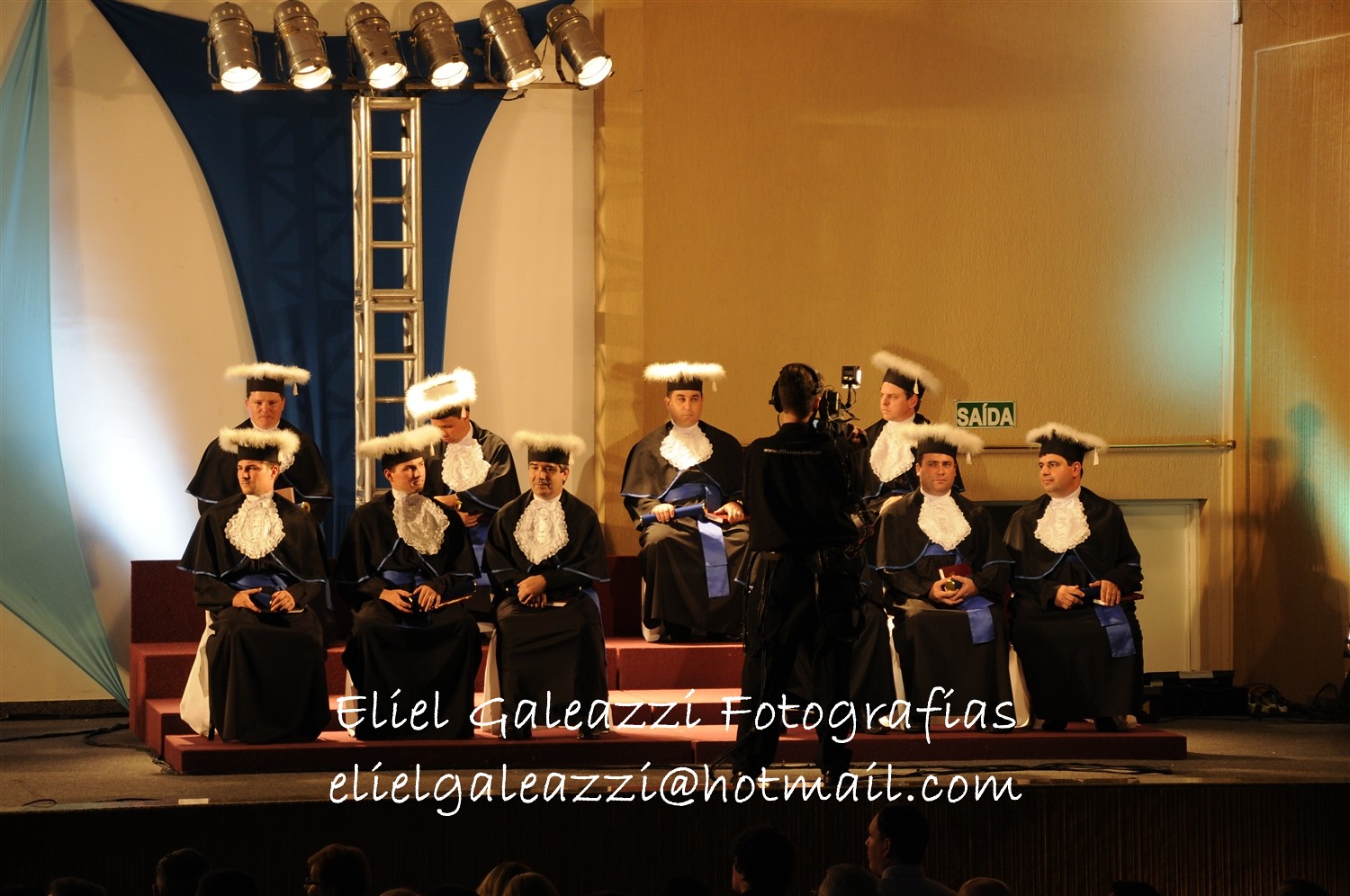This detailed photograph captures an indoor stage scene featuring ten men situated on a wooden bench made of dark-stained wood blocks. There are four men in the elevated back row, and six in the front row, all around middle-aged and appearing to be white males. Each wears a distinctive outfit reminiscent of traditional English judge attire, with long black robes adorned with white borders and complemented by a frilly white chest piece hanging from their necks. Their heads are topped with unique caps that resemble graduation mortarboards, but covered in white fur with a yellow square on top.

In front of these men stands a cameraman, partially obscuring one of the men in the front row. He is intently filming the group, likely for a television program or ceremony. The background of the stage varies, featuring a smooth orangish wall on the right and a white wall on the left, draped with blue fabric. Above, a steel girder supports six spotlights that illuminate the scene. Additionally, the setup includes text reading "Eliel Gazilla Photographs" with the email address "elieligaleaacz@hotmail.com" indicating some form of credit or contact information. The heads of audience members are visible in the foreground, observing the proceedings, lending a sense of a communal ceremonial or formal event.